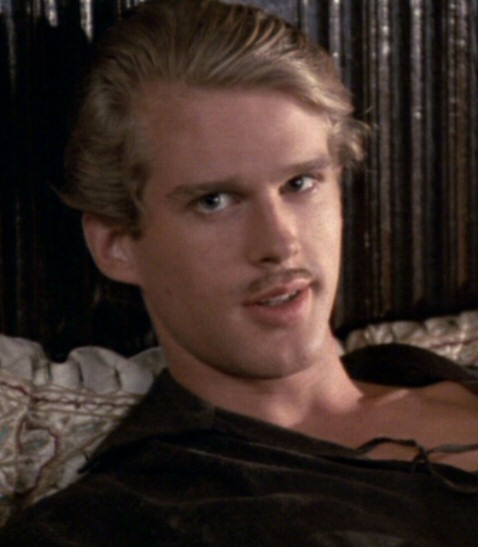This image features a man in his mid-30s with fair complexion and blue eyes, gazing directly at the camera. He sports a blonde mustache and slicked-back, dirty blonde hair. His attire appears to be a dark, possibly velvety, loose-fitting shirt. The man’s slightly open mouth forms a subtle smile. The photo has a grainy, slightly blurry quality, suggesting it may have been taken in the 70s or 80s. The setting suggests he is reclining; the composition includes a white pillow with intricate red, green, gold, and blue stitching, partially visible at the bottom third of the frame. The background consists of a brown headboard or wall, potentially with individual rods or paneling, spanning the top two-thirds of the image.